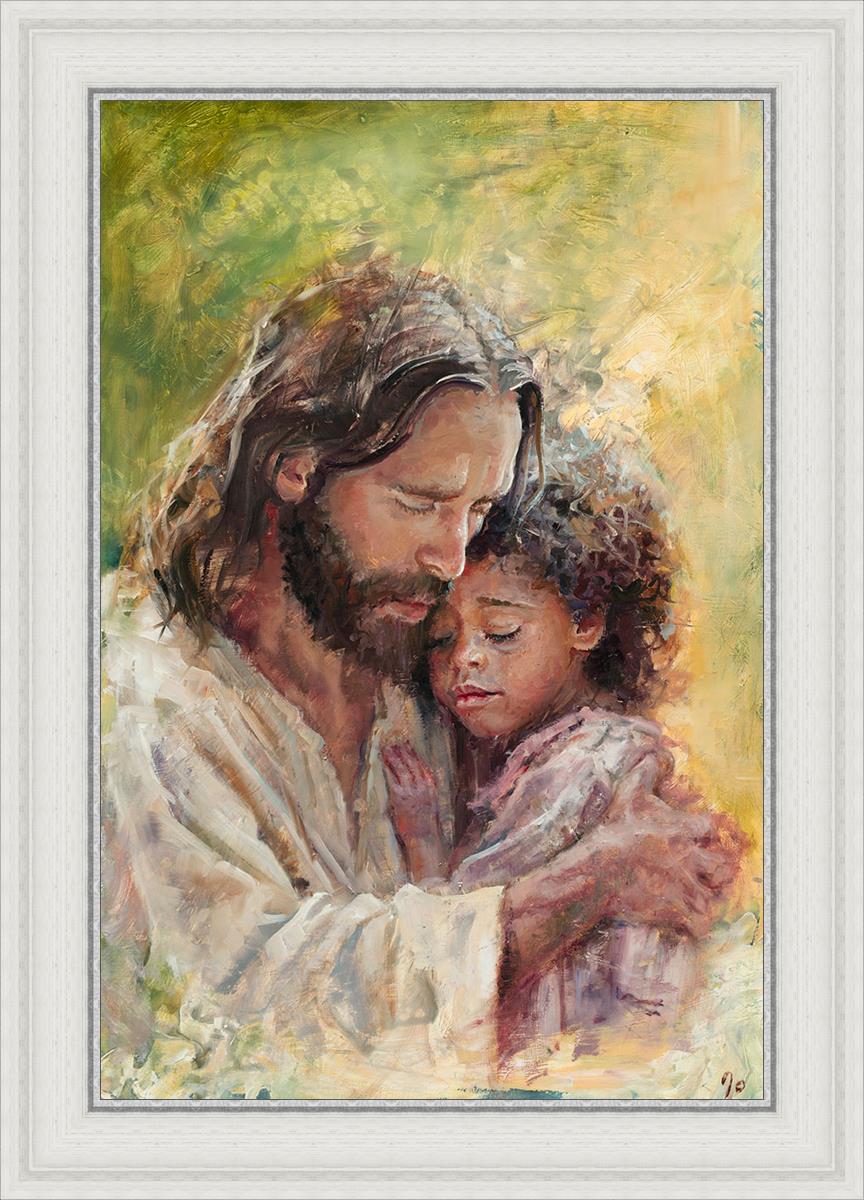This detailed oil painting depicts Jesus, identified by his gentle expression and familiar iconography, holding a small African-American child in a tender, comforting embrace. Jesus is portrayed with shoulder-length wavy brown hair, a brown beard and mustache, and light peach slightly tanned skin. He is dressed in a white robe, consistent with traditional depictions. The child, likely around five years old, has a thick, curly afro and warm brown skin. She is dressed in a pinkish robe and nestles close to Jesus with one hand resting against his chest, both of them with their eyes closed, suggesting a moment of spiritual significance or emotional solace.

The background of the painting features swirling patterns primarily in shades of green and yellow, adding dynamic yet serene energy to the scene. This oil painting is encased within a white, matte-finished wooden frame, which is further accentuated by a thinner light blue border on the inside. The aspect ratio of the painting is taller than it is wide, emphasizing the vertical intimacy of the hug. A mostly illegible, scrawled signature is located in the bottom right corner, attesting to the piece's professional craftsmanship. Despite its abstract details, the use of black, white, various shades of brown, yellow, green, peach, pink, purple, and a touch of red, all contribute to the rich and evocative atmosphere of the artwork.